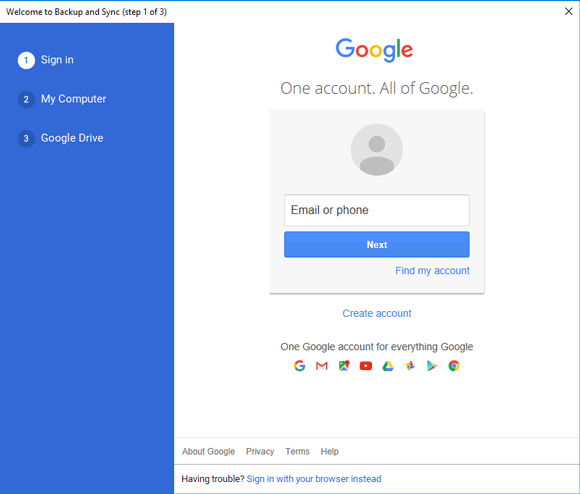In this image, we see a screenshot of the Google Backup and Sync sign-in page for Google email. The header at the top left reads, "Welcome to Backup and Sync, Step 1 of 3." To the top right is an 'X' symbol for closing the window.

Below the welcome message, the screen is divided into three sections:
1. Sign In: Denoted by the number '1' inside a white circle.
2. My Computer: Indicated by the number '2' in a dark bluish circle.
3. Google Drive: Marked by the number '3,' also in a dark bluish circle.

The background of this vertical, rectangular section is a solid blue color.

In the middle of the image, there is a section where users can enter their email or phone number. At the top center, the Google logo appears with its signature colors: blue, red, yellow, blue, green, and red, followed by the text, "One account. All of Google."

Below the input box for the email or phone number, there are buttons labeled "Next," "Find My Account," and "Create Account." Further down, the text reads, "One Google Account for everything Google," accompanied by a row of icons representing Google services such as Gmail, Calendar, YouTube, Google Drive, Google Play, and Google Chrome.